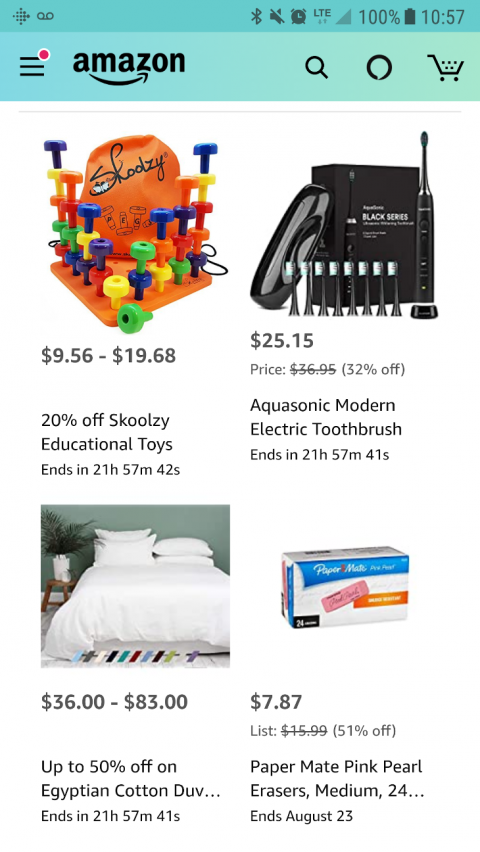**Detailed Caption:**

The image is a screenshot of an Amazon webpage, specifically a wishlist or recommendation section, captured on a smartphone. At the very top, common status bar icons are visible: the Amazon logo is centered, along with indicators for Bluetooth, audio, an alarm set, LTE signal strength, 100% battery charge, and the current time, which reads 10:57. Below the status bar, the Amazon search bar spans the width of the screen, with three horizontal lines on the left indicating a menu, marked by a red dot suggesting a new notification or message.

The main content area displays four recommended items, arranged in a grid format against a white background. In the upper left corner, there's a product labeled "Skoozie," advertised as an educational toy currently on sale for 20% off. To its right is the "AquaSonic Modern Electric Toothbrush," showcasing a sleek design. On the lower left is an "Egyptian Cotton Duvet," likely emphasizing its luxurious and comfortable quality. Adjacent to the duvet on the lower right, a pack of "Paper Mate Pink Pearl Erasers" is featured. The overall layout is clean and uncluttered, focusing on suggested items that the user may find interesting based on their browsing habits.